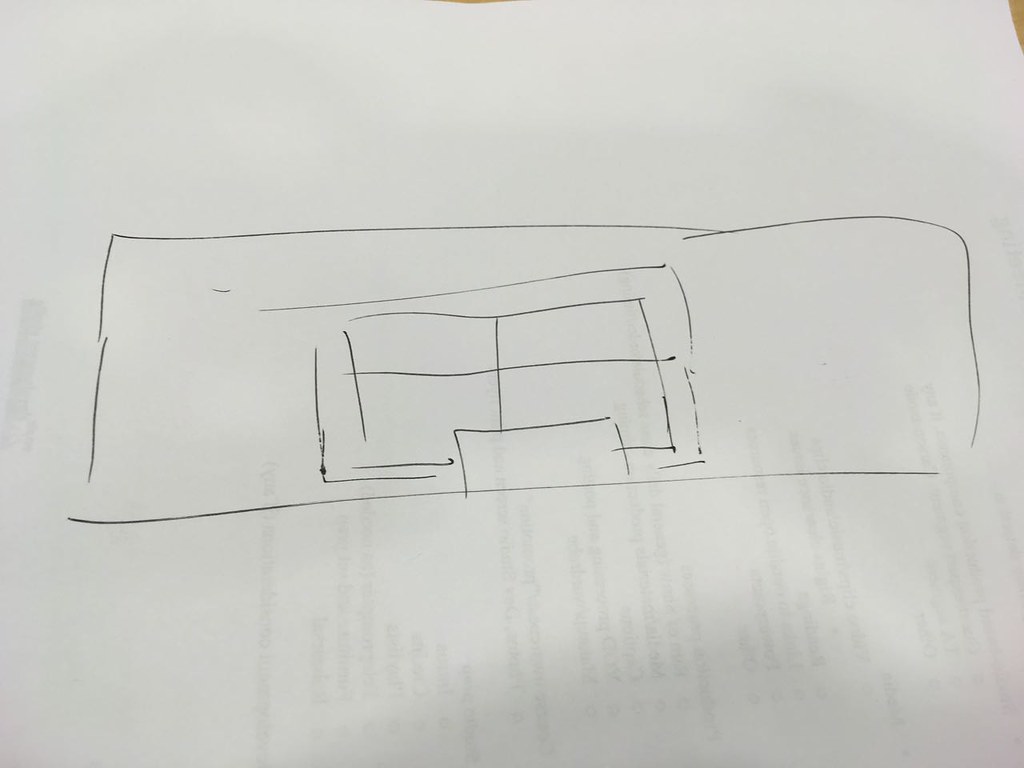Capturing the essence of a preliminary sketch, this image showcases a rough pen line drawing on a sheet of white paper. The drawing occupies approximately one-third of the paper, centered exactly with ample blank space above and below it. The sketch itself consists of a large horizontal rectangle, inside of which is another slightly smaller horizontal rectangle. A cross-like figure within the inner rectangle gives it a window-like appearance. Below this structure, a small additional rectangle, whose purpose is unclear, contributes to the overall composition. The lines of the drawing are not precisely squared off and feature occasional gaps, indicative of an early conceptual stage. There is text visible faintly on the paper, possibly from being printed on the other side or through another sheet underneath. This evokes the sense of an artist's rudimentary sketch, likely drawn vertically but presented horizontally.